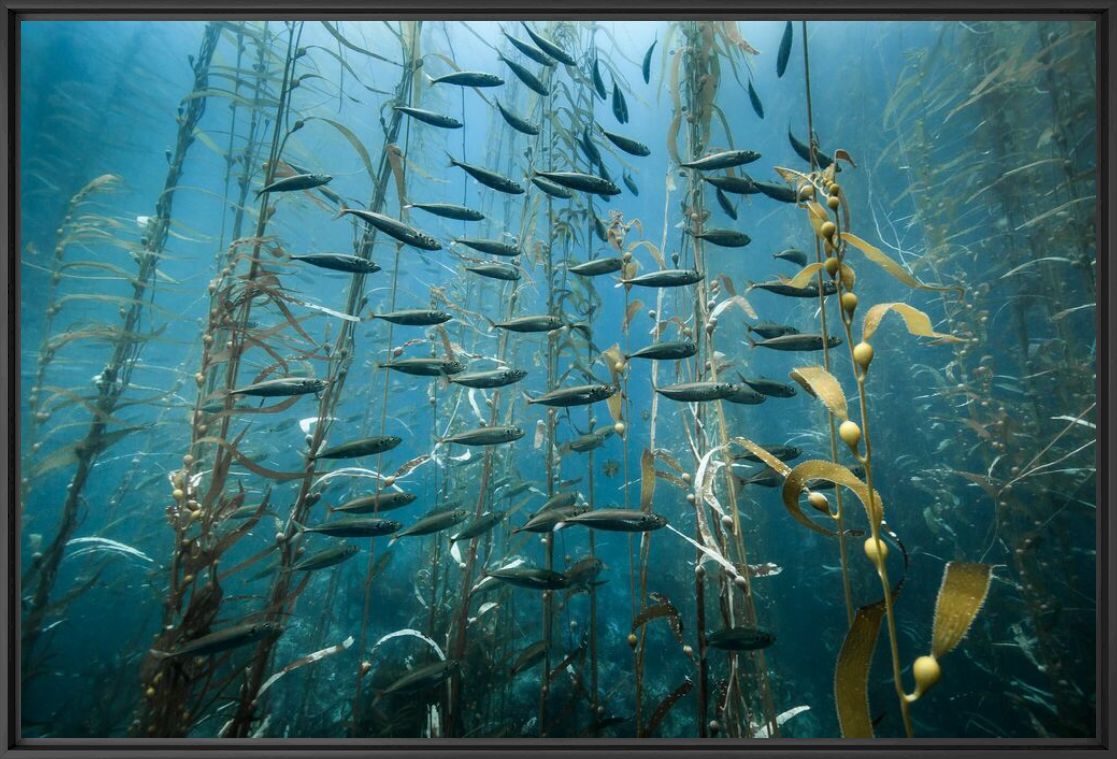This horizontally aligned, rectangular photograph, bordered by grey-black-grey stripes on all sides, captures an enchanting underwater scene suffused with sunlight filtering down from the surface. Central to the image, slightly towards the left, natural light illuminates the vivid blue water, revealing a bustling kelp forest teeming with life. The slender, gray fish, about 1.5 centimeters long, swim predominantly from left to right, but some venture in various directions, primarily visible in the middle third of the scene.

In the foreground on the right, a yellowish-brown kelp frond stretches about 8 centimeters high, its wavy leaves adorned with tiny hairs and buoyant bulbs tethered to the stalk. Towards the left middle, another kelp stalk stands out with its reddish hue, contrasting with the predominantly blue and green palette of the seascape. The delicate interplay of light and water paints a serene, lifelike underwater tableau, making this image appear as if it belongs in a scientific magazine.